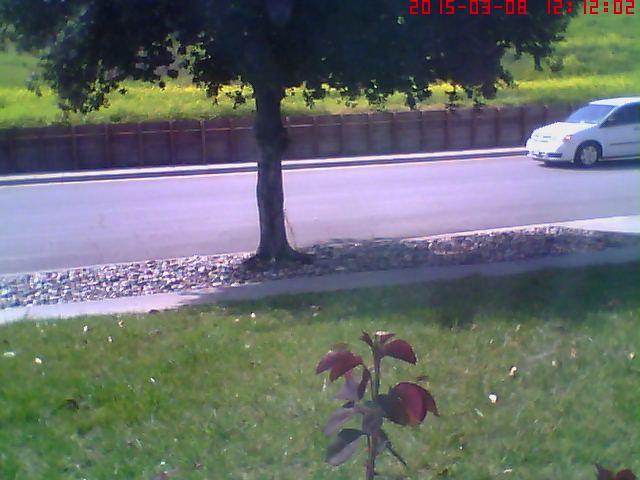This photograph, taken from the interior of a residential home, offers a scenic view of the front yard, sidewalk, and road. In the foreground, a tall plant with dark red leaves decorates the scene, leading the eye across the vibrant green grass of the front lawn. Adjacent to the lawn, a narrow cement sidewalk runs parallel to the road.

Between the sidewalk and the road lies a landscaped stretch filled with an assortment of rocks and pebbles, where a large, full leafy tree stands as a centerpiece. The paved road beyond hosts a solitary white car traveling from right to left.

On the far side of the road, another sidewalk borders a brown wooden fence, behind which a lush green grassy hill rises, adding depth and a touch of nature to the picturesque suburban setting.